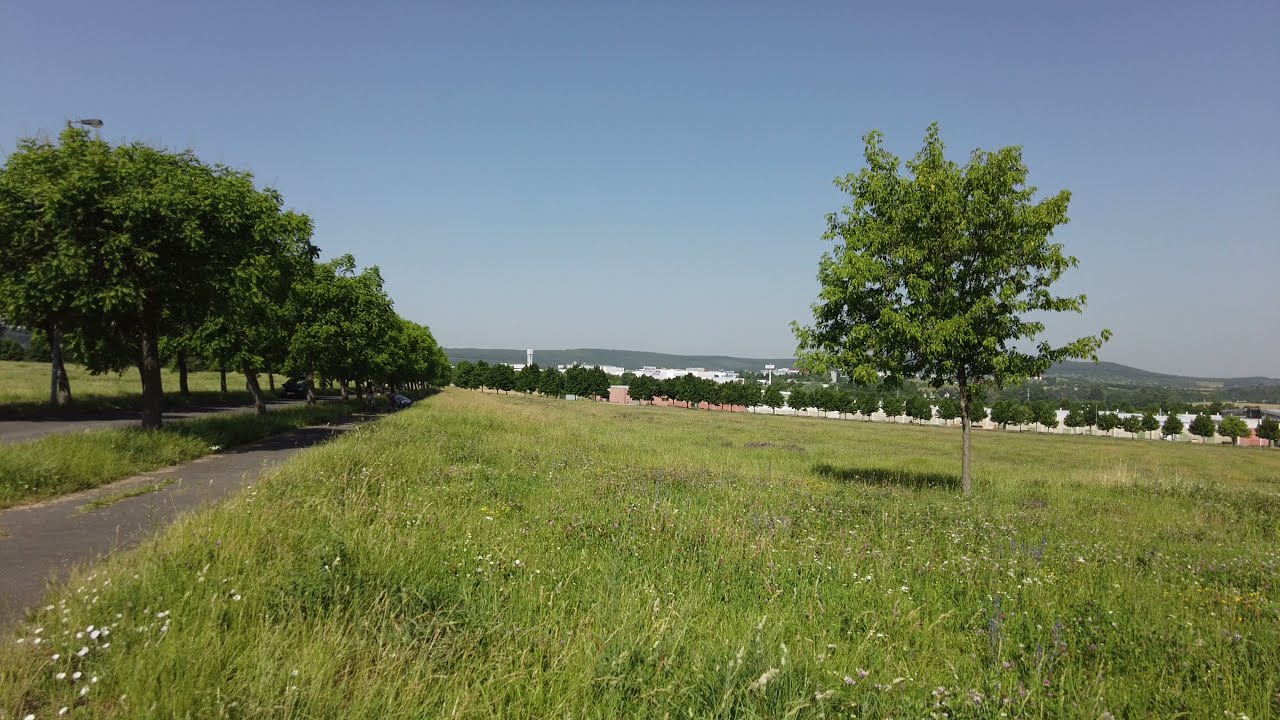This daytime landscape photograph captures an expansive, green field meadow under a pristine, blue, cloudless sky. A tree-lined path occupies the left third of the image, extending from the foreground to the distant horizon. In contrast, the right third of the image features a solitary, small-trunked green tree or shrub. The lush, uncut grass stretches across the foreground, with individual blades clearly visible. The background presents a low, flat hillside with a tree-lined perimeter. There are no sun flares, wildlife, people, vehicles, or buildings visible, contributing to a serene and undisturbed rural scene. The distant horizon is marked by a horizontal line of trees, and subtle, small white structures appear sporadically behind the single tree on the right, adding a touch of intrigue to the otherwise clear and tranquil landscape.